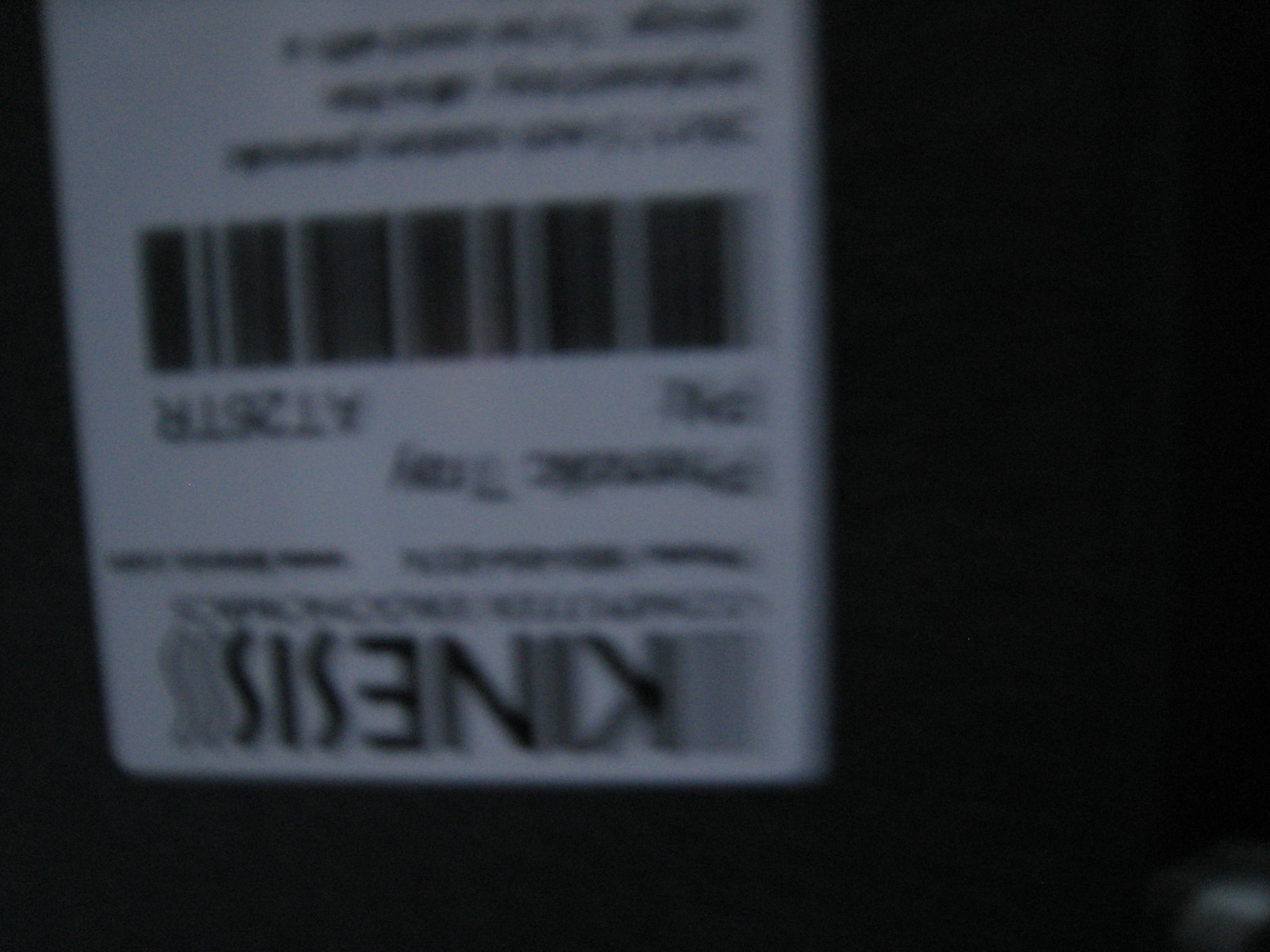This image is a blurry, out-of-focus photo with a black background, capturing a rectangular white label affixed to an indistinguishable black object. The label is positioned near the upper left to center of the image and appears to be upside down. In bold black letters at the top of the label, it reads "K-I-N-E-S-I-S." Below this, there is smaller black text, including a product number and additional writing, all predominantly illegible due to the poor quality of the photo. A barcode is situated beneath this text, with further writing underneath it, also blurred and smudged, making it difficult to decipher. The overall dark and unclear nature of the image suggests the photo was taken hastily or with a moving camera.